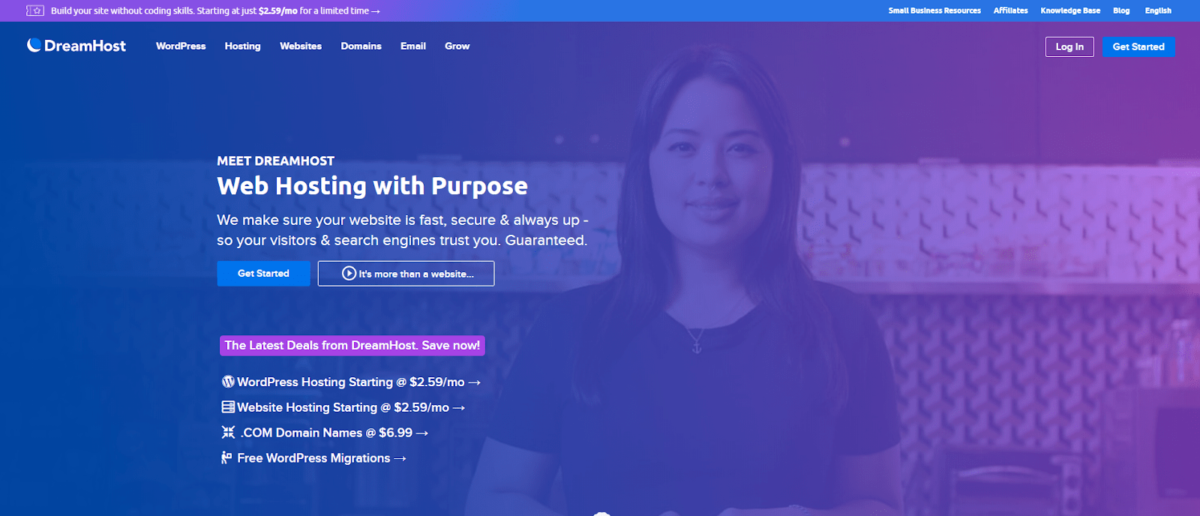This image is a promotional screenshot from the DreamHost website, featuring a clean and modern design with a blue-to-dark-purple gradient background. The gradient transitions smoothly from blue on the left side to purple on the right. 

At the top of the screen, a prominent banner reads: "Build your site with coding skills starting at just $2.59 a month for a limited time." 

In the middle of the screen, there is an image of a woman with long dark hair, wearing a dark t-shirt and a necklace featuring a ship's anchor. To her right, bold text highlights DreamHost's mission: "Meet DreamHost, web hosting with purpose. We make sure your website is fast, secure, and always up so your visitors and search engines trust you—guaranteed."

Beneath this section, there are two options encouraging users to "Get Started." Additionally, a subheading below reads: "More than a website," leading into the latest deals from DreamHost. 

Further information outlined includes:

- WordPress hosting starting at $2.59 a month
- Website hosting starting at $2.59 a month
- .com domain name at $6.99
- Free WordPress migrations

These options are presented with clickable elements for easier navigation. The overall aesthetic of the page combines visual appeal with clear, actionable information.